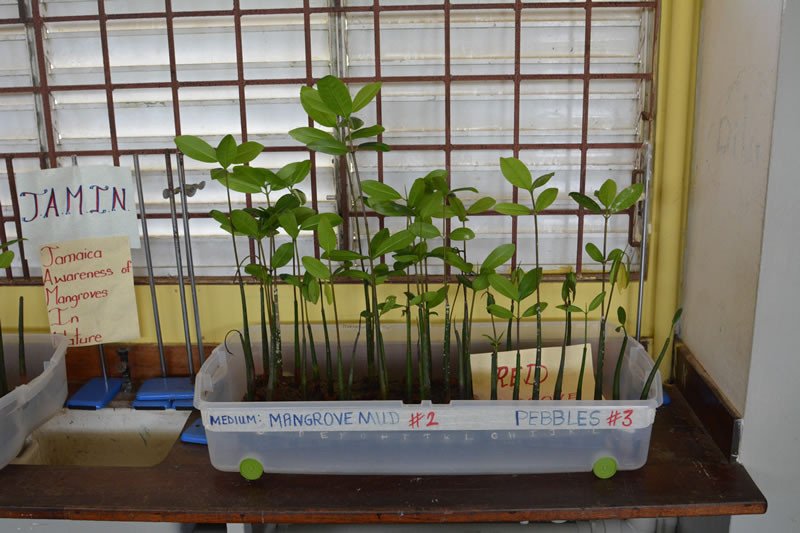This indoor image features a room with a prominent yellow back wall and white side walls. A vertical pipe runs up the right side of the image, and a window with white shades is covered by protective metal bars, likely bronze-colored, set within a yellow frame. A dark red wooden table is placed against the yellow wall. On this table sits a clear, rectangular plastic box filled with black dirt and labeled with tape that reads "medium mangrove mud number two" and "pebbles number three." Emerging from the soil inside the box are green stems of varying heights, each adorned with similar green leaves. Additionally, there is a sign on the plastic box that explains the display: "Jamin, Jamaica awareness of mangroves in nature," indicating that the bars on the window are likely for security purposes due to the location in Jamaica.